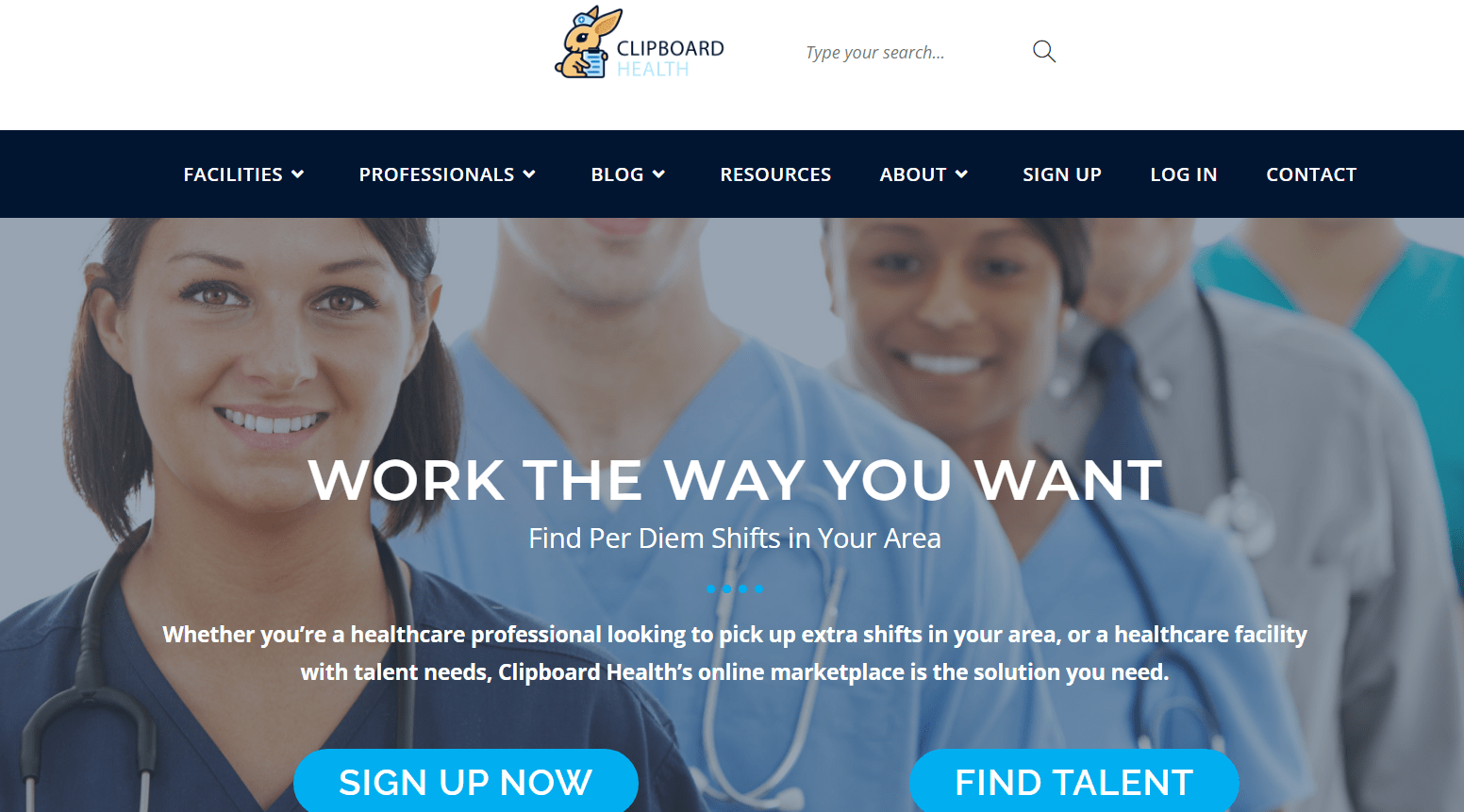This horizontally-oriented image features a detailed interface from a website for Clipboard Health. Dominating the top portion of the image, there's a small icon resembling an orange rabbit holding something blue, accompanied by the website's name "CLIPBOARD" in black, capital letters, and "Health" below it in turquoise. Adjacent to this is a search bar with a magnifying glass icon. The very top section, in a horizontal rectangular area either navy blue or black, displays the menu options in white, all capital letters: Facilities, Professionals, Blog, Resources, About, Sign Up, Log In, and Contact.

In the background, a muted image depicts five individuals, likely healthcare professionals, with two confirmed to be women (the first and third) and one man (the fourth). These figures are garbed in blue surgical outfits with V-necks, many adorned with stethoscopes over their shoulders or around their necks.

Central to the image, large white capital letters state "WORK THE WAY YOU WANT," with a smaller white font below that reads, "Find Per Diem Shifts In Your Area." Beneath this text, there are four turquoise dots followed by another white text block: "Whether you're a healthcare professional looking to pick up extra shifts in your area or a healthcare facility with talent needs, Clipboard Health's online marketplace is the solution you need."

At the bottom of the image, there are two horizontally-aligned turquoise ovals with white capital lettering. The first oval, on the left, says "SIGN UP NOW," while the second oval, on the right, reads "FIND TALENT."